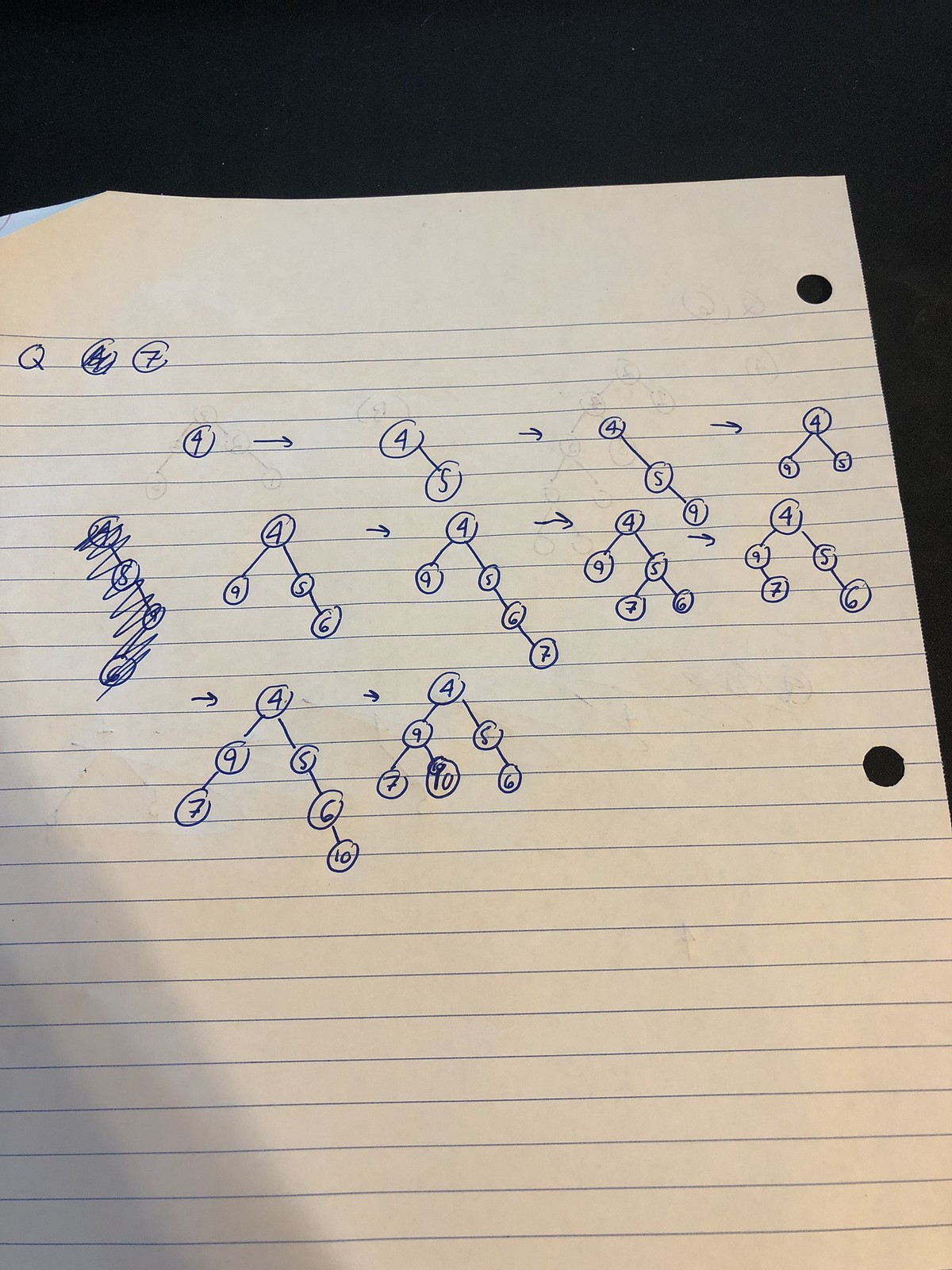The image features a black background that appears to be a black table or desk, highlighting a white, regular lined piece of notebook paper. This paper, designed for a spiral binder, has its punched holes on the right side, suggesting we are viewing the back of the page. The paper is semi-transparent, revealing handwritten diagrams in blue ink on both sides. 

The diagrams consist of a series of interconnected numbers, forming potentially mathematical theorems or equations. The sequences primarily involve the numbers 4, 5, 6, 7, 9, and 10, each circled or enclosed in shapes reminiscent of billiard balls on a pool table.

- The first diagram shows the number 4 connected by arrows to another 4 and then from 4 to 5 diagonally. 
- The second diagram follows with 4 leading to 5, then 5 to 9.
- The third diagram creates a triangular shape with 4 linking to 5 and 9.
- The fourth diagram shows a connection from 4 to 9, a separate line from 4 to 5, and from 5 to 6.
- The fifth diagram extends the sequence to include 6 going to 7.
- The sixth diagram, similar to earlier ones, has the 4 connected to both 9 and 5, with 5 branching to 7 and 6.
- The seventh diagram also follows the pattern with 4 connecting to 9, then 7, and from 5 to 6.
- The final diagram on this side illustrates a more complex sequence: 4 to 9, then 9 to 7, 4 to 5, 5 to 6, and finally 6 to 10. Then comes the ultimate diagram with 4 to 9 and 5, with 9 branching to 7 and 10, and 5 branching to 6.

The complexity of these numbered sequences, primarily revolving around the number 4, suggests an attempt to solve an equation or theorem. Despite the intricate penmanship, the exact mathematical purpose remains ambiguous.